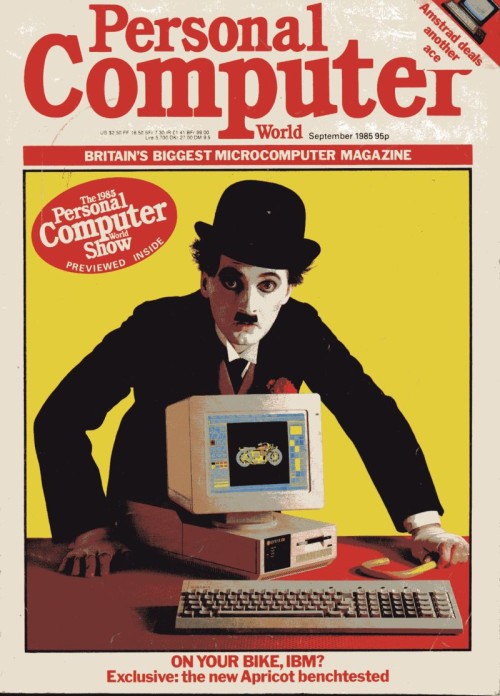This is a vertically aligned cover of the magazine "Personal Computer World" from September 1985, priced at 95p. The background gradient transitions from light tan at the bottom to white at the top. The title "Personal Computer World" is prominently displayed in large red letters at the top, with "Personal" being smaller and "World" even smaller. To the right of "World," the issue details are mentioned: "September 1985 95P". 

Central to the cover is an eye-catching, square image of a man dressed as Charlie Chaplin. He wears a black suit jacket, a black hat, and has a tiny black mustache, with his face painted white. This intriguing character is standing in front of an old, tan-colored computer displaying a motorcycle on its screen, with a similarly colored keyboard in front. The computer rests on a red table and is set against a solid yellow background.

Additionally, there is a noticeable speech bubble to the man's left, shaded in red with white text that reads, "The 1983 Personal Computer World Show Previewed Inside." At the bottom of the cover, there's another significant banner stating, "On Your Bike IBM Exclusive: The New Apricot Bench Tested."

Incorporated subtly within the design, the subtitle declares the publication as "Britain’s Biggest Microcomputer Magazine," reaffirming the magazine’s stature during that period.